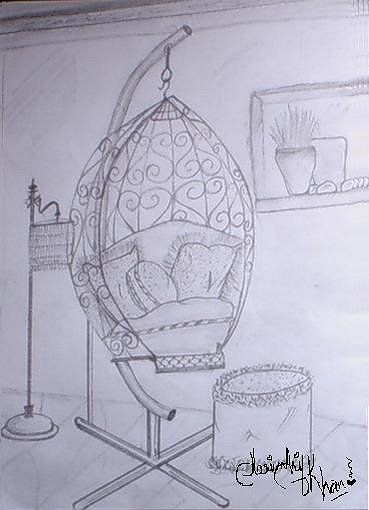This detailed pencil drawing centers around a hanging egg-shaped chair. Suspended by a hook at the top, the chair's frame resembles a letter C sitting on an X-shaped base. The incomplete frame and legs give it an open, airy feel. The chair is adorned with a cushion and three pillows, and its intricate design features heart-shaped patterns on the back and sides, with the tops of the hearts curling inward to form small half circles.

Directly in front of the chair sits a tall, cylindrical ottoman, decorated with a fuzzy texture on both the top and bottom. Behind the chair, to the left, there appears to be a birdcage-like structure adding to the room's decor. On the right, a little above the chair, a square shelf is built into the wall, holding a planter and a small rectangular object.

A floor lamp with a curved post and a plaid lampshade stands behind the chair, its round base visible on the floor. The floor itself is depicted with lines, suggesting wooden boards, which adds a rustic touch. The top and bottom edges of the drawing have shading, lending a sense of depth and framing to the scene.

In the upper right-hand corner, there's a window with a pot of vegetation and an adjacent square object. The drawing also showcases a darkly shaded ceiling with ceiling molding details. In the lower right-hand corner of the sketch, the artist's signature appears along with a small heart emitting smoke, although the signature is not legible. Overall, the artwork captures a cozy and eclectic interior scene with meticulous attention to texture and design elements.